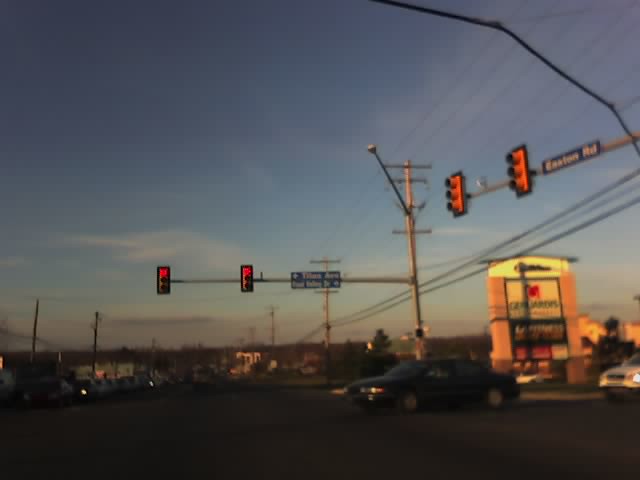This blurry photograph captures a suburban intersection from the perspective of a car stopped at a red light. Dominating the center of the image are two red stoplights, and on the right-hand side, there are two additional stoplights with unreadable colors. The stoplight on the right features a street sign reading "Easton Road," while the middle stoplight points directions to the left and right. The sky, occupying the top 75% of the image, is a light blue with scattered wispy clouds, punctuated by telephone poles and wiring stretching across the scene. 

The intersection is busy, with two cars—a black sedan and a white or silver SUV—pulling out, presumably having received a green light. In the opposite lane, a line of cars queues up, waiting at the intersection. A classic suburban shopping center sign stands prominently on the right side, showcasing multiple stores, although its details are blurred and not legible. The lighting suggests it’s around sunset, as the sun still illuminates the top of the shopping center sign while the road below lies in shadow.